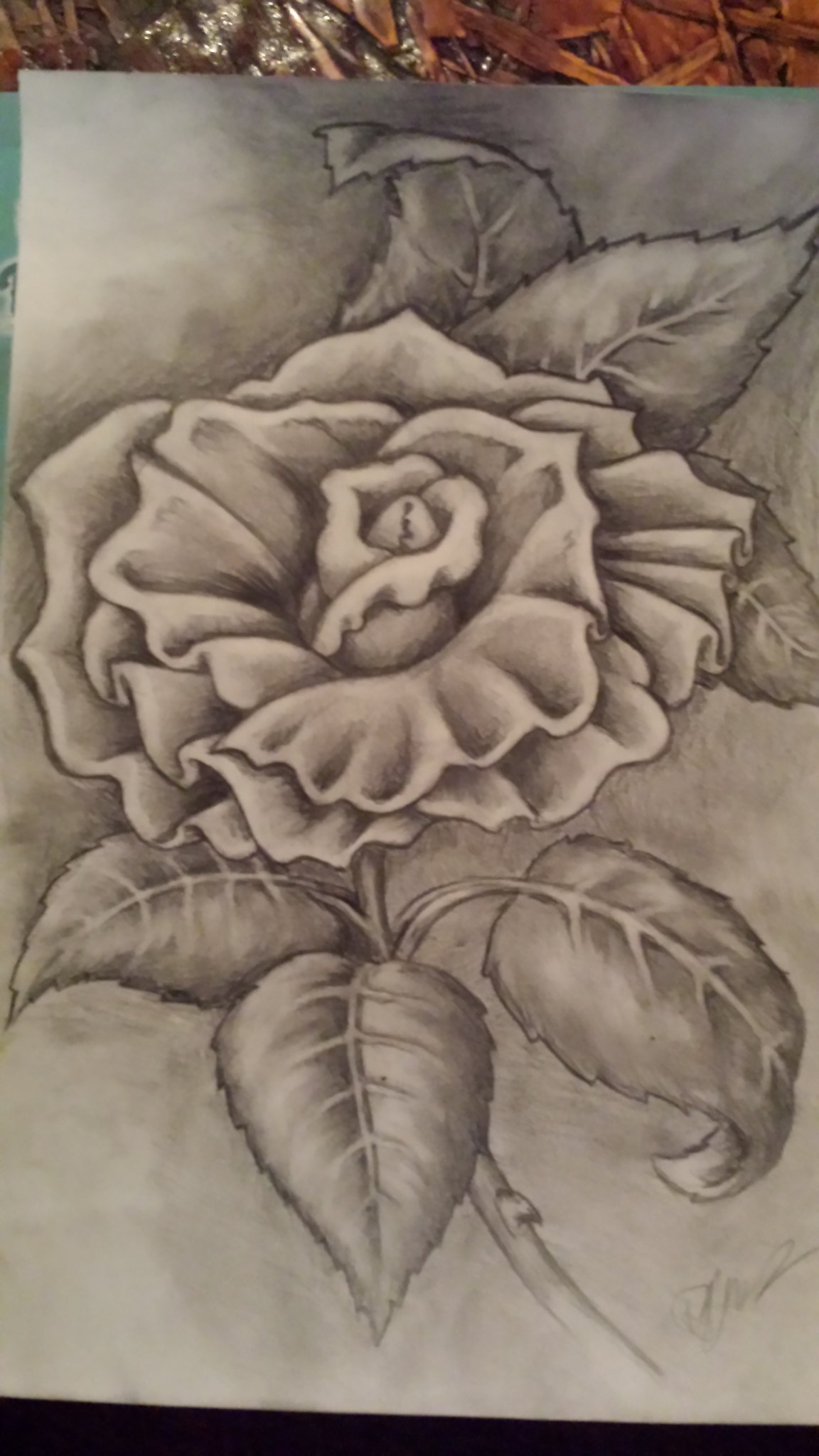This image is a close-up photograph of a detailed graphite drawing of a single rose. The rose itself is the central focus, characterized by intricate shading and blending on the petals and the clusters of leaves that surround it. The drawing features leaves at both the top and bottom, with some curling and others appearing more rigid. The stem of the flower is visible and includes at least one thorn, adding to the realism. A signature is placed in the bottom right corner; however, it is not fully legible. The drawing appears to have a distinctive, almost prison art vibe, making it reminiscent of a tattoo design. The background behind the flower has additional shading, though it is unclear if this represents a shadow or merely a backdrop. The piece of paper with the drawing is laid on a textured surface, and the photo seems to be taken slightly from above, likely with a cell phone.